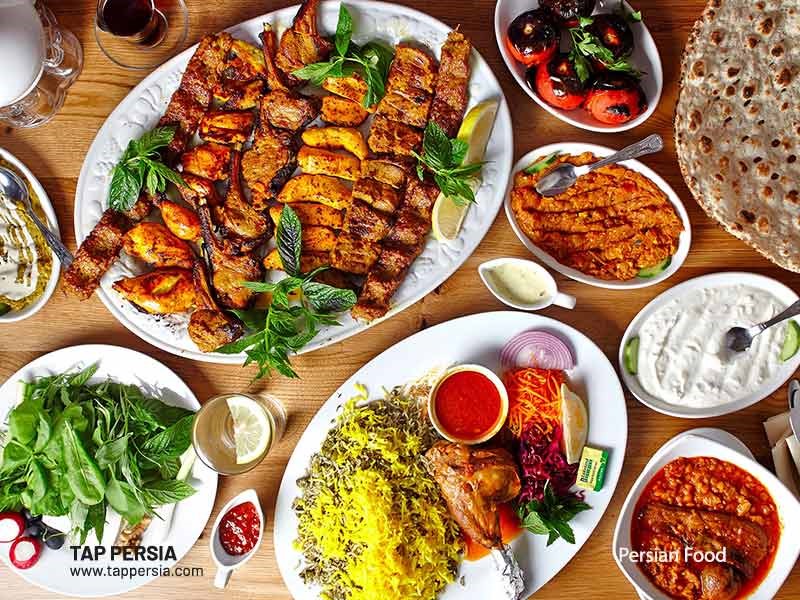The top-angle photograph, likely from a food blog or page, captures a sunlit wooden table adorned with a diverse and appetizing array of dishes. At the forefront, multiple kebab plates showcase golden-brown grilled chicken, shrimp, bacon, and other meats, garnished with basil leaves and lemon wedges. A prominent plate displays a serving of vibrant yellow pilaf or rice, accompanied by large mutton leg pieces, red sauce, onion slices, lemon slices, a butter packet, and garnishes including basil leaves, beetroots, and carrot slices. Towards the left, another significant plate holds a medley of veggies, potentially with a chicken pie, encircled by several smaller bowls containing red and white sauces, grilled tomatoes, leafy spinach or salad greens, and a yogurt-like dish. Adding to the assortment, a basket of Indian bread (roti or naan), a jug, and various glasses, including one with water and a lemon slice, also adorn the table. The scene is polished off with watermarks from teppersia and identifying it as Persian food.